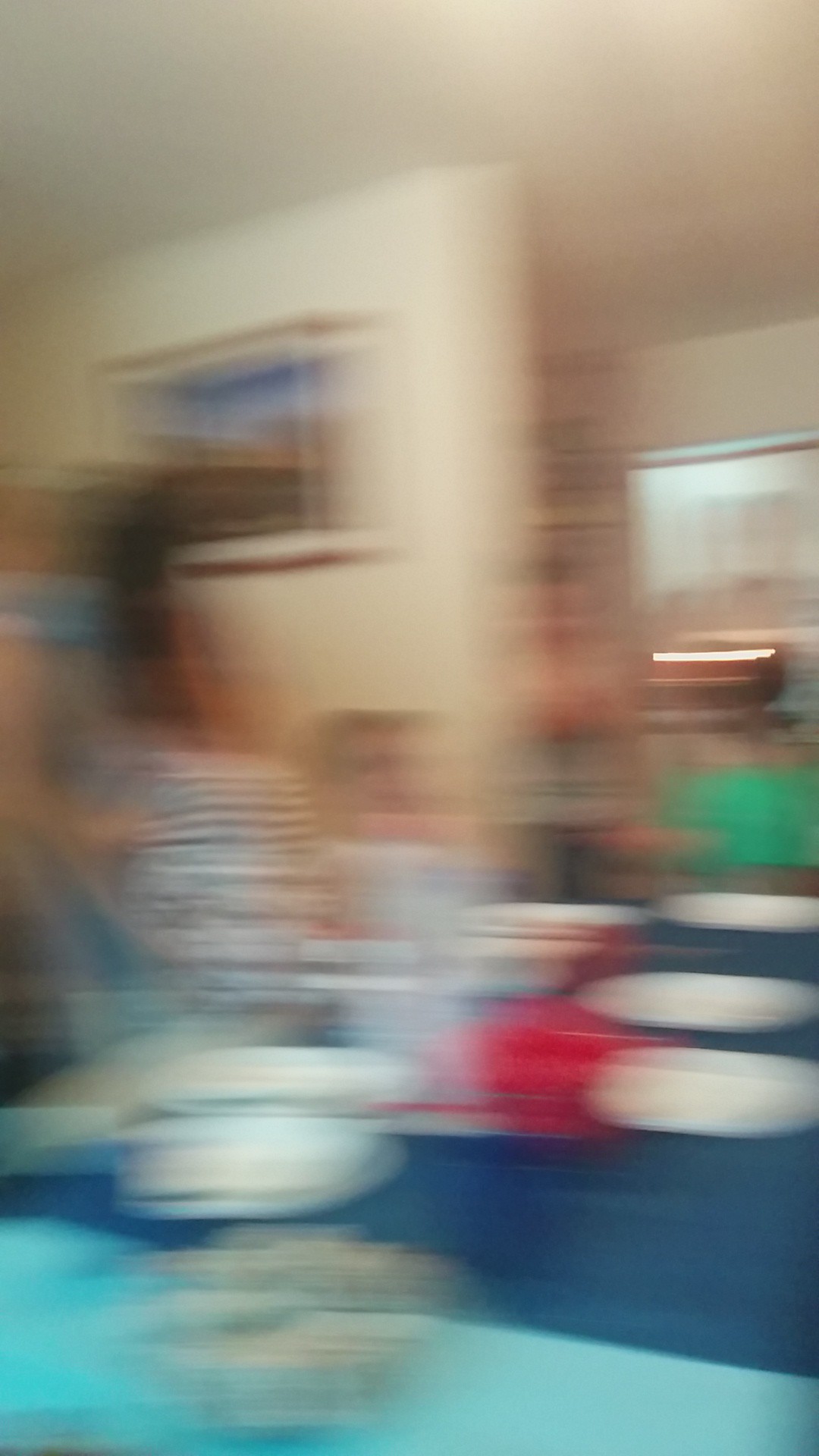This is a color photograph characterized by significant blurriness and lack of focus, making precise identification challenging. The image seems to depict a scene that possibly includes a kitchen counter. The counter, if present, showcases two distinct shades of blue: a light turquoise stripe in the bottom left-hand corner, and a royal blue color dominating the remaining visible surface. Scattered across the counter are three objects that appear to be white plates, along with another object that resembles a white bowl. Beyond this counter, a wall and ceiling come into view, both bathed in a very faint golden yellow hue, adding a warm tint to the overall composition.